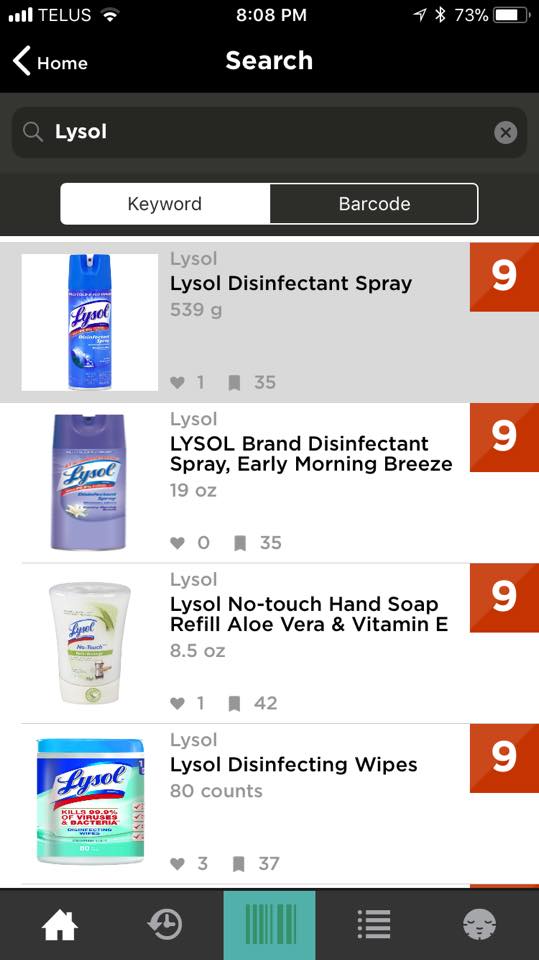This is a detailed screenshot from a smartphone displaying a search for "Lysol" products on a retail app. 

At the top of the screen, several status icons are visible: signal strength bars and the carrier name "TELUS" on the left, then another signal bar, the time "8:08 PM," and to the right, a collection of icons including the battery indicator showing 73%.

Just below this status bar, there's a navigation row with the bolded label "Search" on the right and "Home" on the left, next to a left-pointing caret. Underneath, a search bar displays the query "Lysol" in white text. Below the search bar are two selectable tabs: "Keyword" (which is highlighted) and "Barcode."

The main content showcases four Lysol products:

1. **Lysol Disinfectant Spray (Blue Can)**: 
   - Description: "Lysol disinfectant spray, 539 grams"
   - Engagement: 1 heart, 35 likes
   - Promotion: An orange box with the number 9 to the right of the item

2. **Lysol Disinfectant Spray (Dual Purple Package)**:
   - Description: "Lysol brand disinfectant spray, early morning breeze, 19 ounces"
   - Engagement: 0 hearts, 35 likes
   - Promotion: An orange box with the number 9 to the right of the item

3. **Lysol No-Touch Hand Soap Refill**:
   - Description: "Lysol no-touch hand soap refill, aloe vera and vitamin E, 8.5 ounces"
   - Engagement: 1 heart, 42 likes
   - Promotion: An orange box with the number 9 to the right of the item

4. **Lysol Disinfecting Wipes (Light Blue Canister)**:
   - Description: "Lysol disinfecting wipes, 80 count"
   - Engagement: 3 hearts, 37 likes
   - Promotion: An orange box with the number 9 to the right of the item

At the bottom of the screen, there are five icons representing different navigation options: home, clock, barcode, list, and a circle resembling a sleeping moon.